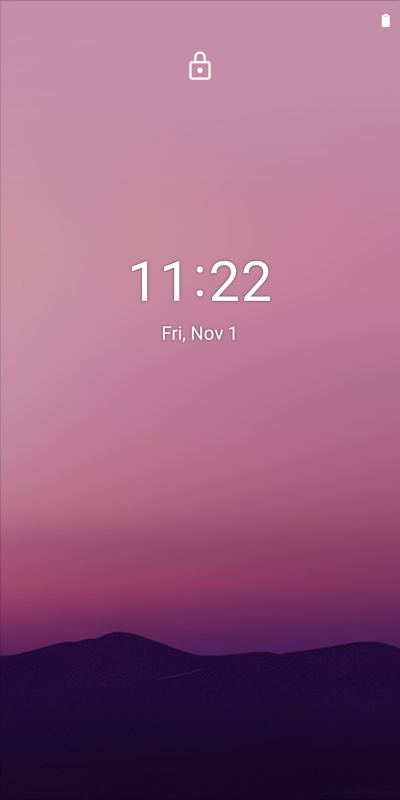The image features a gradient purple sky that darkens towards the horizon. In the top right corner, a thin white line is visible. Centered at the top of the image, a white icon resembling a lot is prominently displayed. Beneath this icon, in large white letters, the time "11:22" is clearly shown. Directly below, in smaller white letters, the date is formatted as "FRI, NOV 1." The lower part of the image depicts black mountains or gently rolling hills, devoid of any discernible features, suggesting it was taken at a very dark time of the day. The sky is void of additional text, symbols, emojis, defects, colors, wildlife, stars, people, or animals, presenting a clean and minimalist scene.